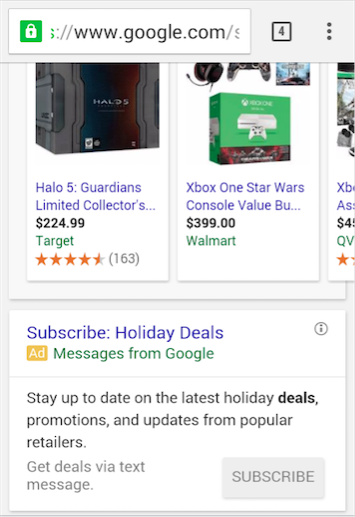Screenshot of a Google search page displaying holiday deals on video game products, captured while zoomed in likely due to an accessibility setting increasing text size. The URL at the top shows Google.com, indicating the search origin. The page shows multiple open tabs and various listed products, including:

1. **Halo 5: Guardians Limited Collector's Edition** – Priced at $224.99 and available at Target.
2. **Xbox One Star Wars Console Value Bundle** – Priced at $399 and available at Walmart.
3. An **Xbox game**, presumed to be **Assassin's Creed**, priced in the $40 range but the full price is cut off along with part of the vendor’s name, assumed to be QVC.

Below the product listings is a Google advertisement promoting holiday deals. The message encourages users to stay updated on the latest holiday deals, promotions, and updates from popular retailers by subscribing to receive deals via text message. An information icon is situated at the top right corner of the advertisement box. The entire page displays in light mode with a bright white background.